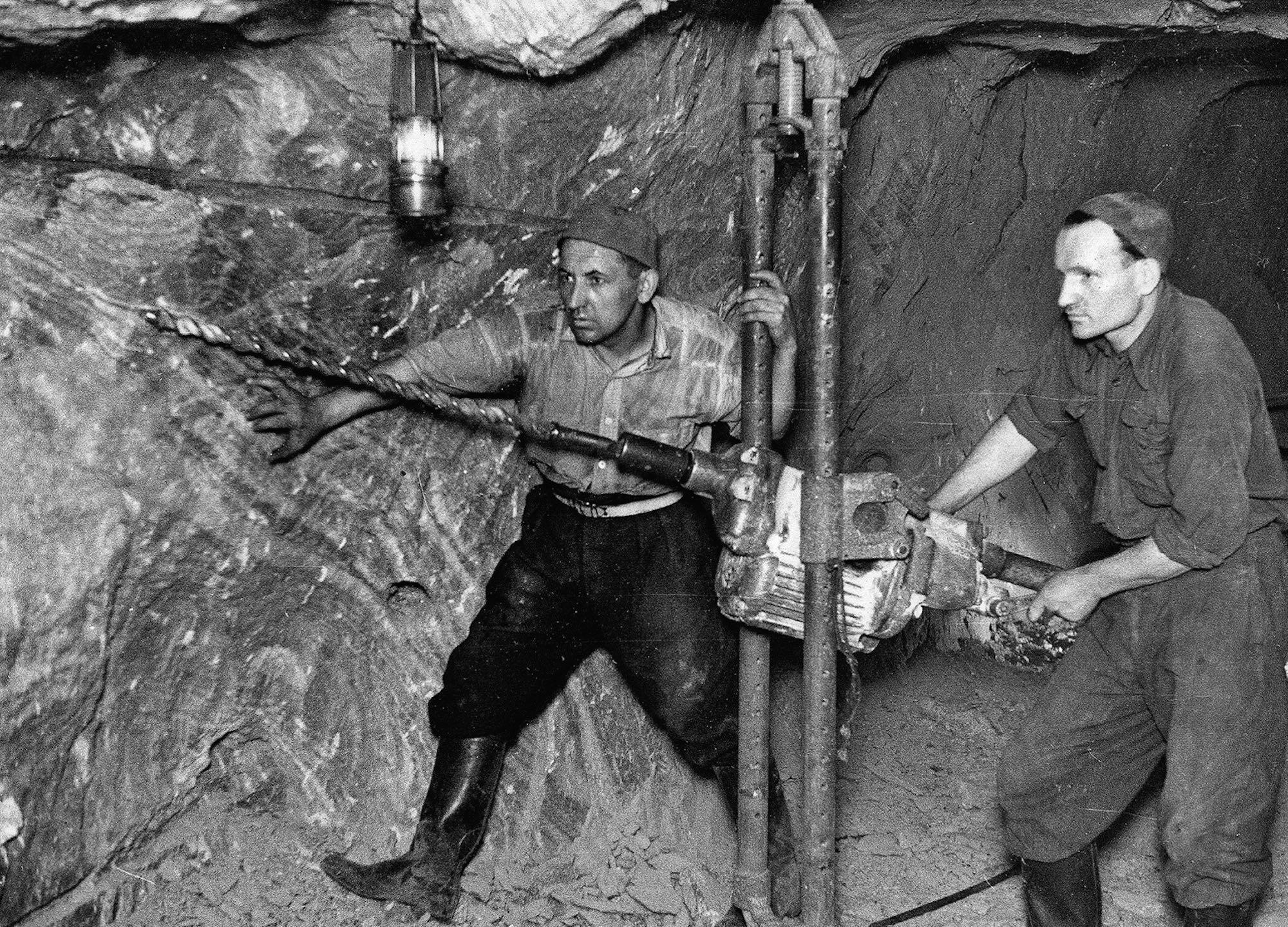In this black and white photograph, set in what appears to be an old mine shaft or underground cave, two men are working diligently amidst their rugged surroundings. The scene is illuminated by a metallic lantern hanging above the man on the left, casting a small but noticeable glow. The men are positioned beside a structure that resembles a stability column, extending from the ground to the ceiling, presumably to support the mine roof. 

The man on the left is dressed in a dirty t-shirt, dark pants, and boots, and wears a cap. His hands, covered in dirt and soot, grip the column, and he is guiding a very long, approximately six-foot drill that is supported by this central structure. The man on the right is wearing a lighter, possibly tan-colored jumpsuit and is actively controlling the handle of the hefty power tool, which features a large drill point at the end.

Surrounded by stone and the debris that typically characterizes a mine, the men’s attire—work clothes, including plaid shirts, belts, dark pants, rubber boots, and caps—accentuates their roles as laborers toiling in a harsh and dirty environment. The drill they are operating appears to be attached to a white machine that aids in its operation. This detailed tableau captures a gritty snapshot of the miner's life and labor underground.